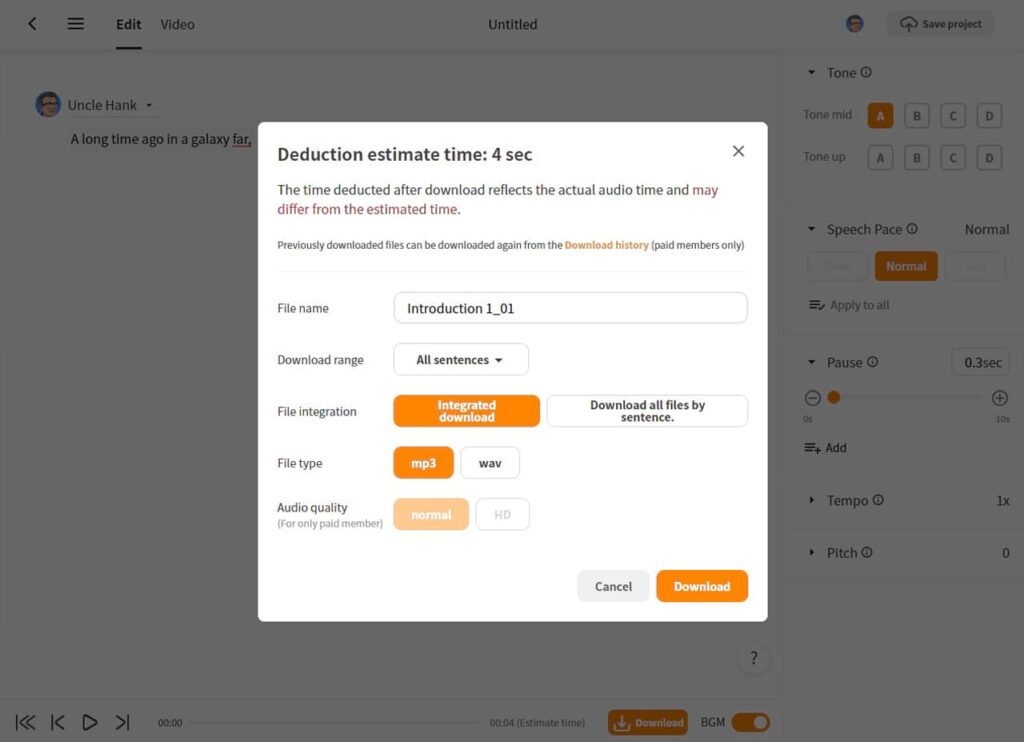This image displays a detailed screenshot of a website interface centered around downloading audio files. The focal point of the screenshot is a prominent white square overlaying the background screen.

In the upper left corner of the white square, there’s a header titled “Deduction Estimate Time for Sections”. A note follows, stating that "The time deducted after download reflects the actual audio time and may differ from the estimated time."

Beneath this, in smaller black text, it reads: “Previously downloaded files can be downloaded again from the download history, available for paid members only.”

Further down, there’s a section labeled "File Name" followed by a white input box containing the text "Introduction_01."

Next, there’s a section titled "Download Range" featuring a dropdown box set to "All Sentences."

Following this is the "File Integration" section, which contains two buttons: an orange button labeled "Integrated Download" and a white button labeled "Download All Files by Sentence."

Below these options lies the "File Type" section, where users can choose between MP3 and WAV formats. The MP3 option is highlighted in orange.

Lastly, the "Audio Quality for Paid Members Only" section offers two choices—Normal and HD—with "Normal" highlighted.

The interface is clearly designed with comprehensive options for users, especially those with paid memberships, ensuring flexible and high-quality audio file downloads.